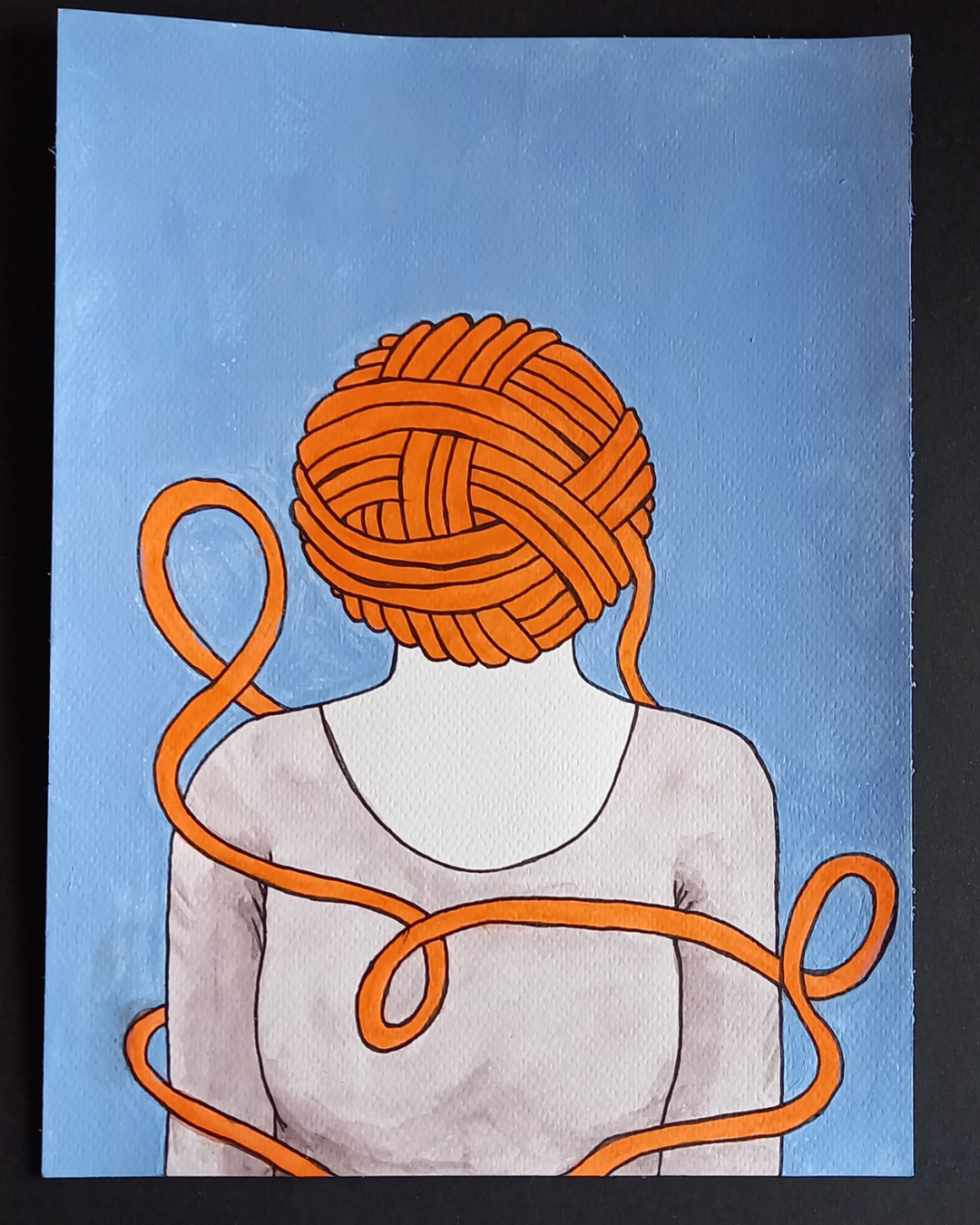The image is a detailed photograph of a painting, rectangular in shape with the longer vertical side. The painting is rendered on a clear-textured canvas or towel paper, featuring a light blue background. Central to the composition, we see a feminine figure, identified as a woman by the presence of breasts and a low-cut, light gray blouse revealing a white neck. The most striking aspect of the painting is the unique portrayal of the woman’s head, which is replaced by an orange ball of yarn. The yarn is intricately wrapped around her body, emerging from her left ear and following a complex path—twisting and turning across her chest, over her shoulders, and around her arms. There is no text present in the image, allowing the intricate and whimsical design to stand out.